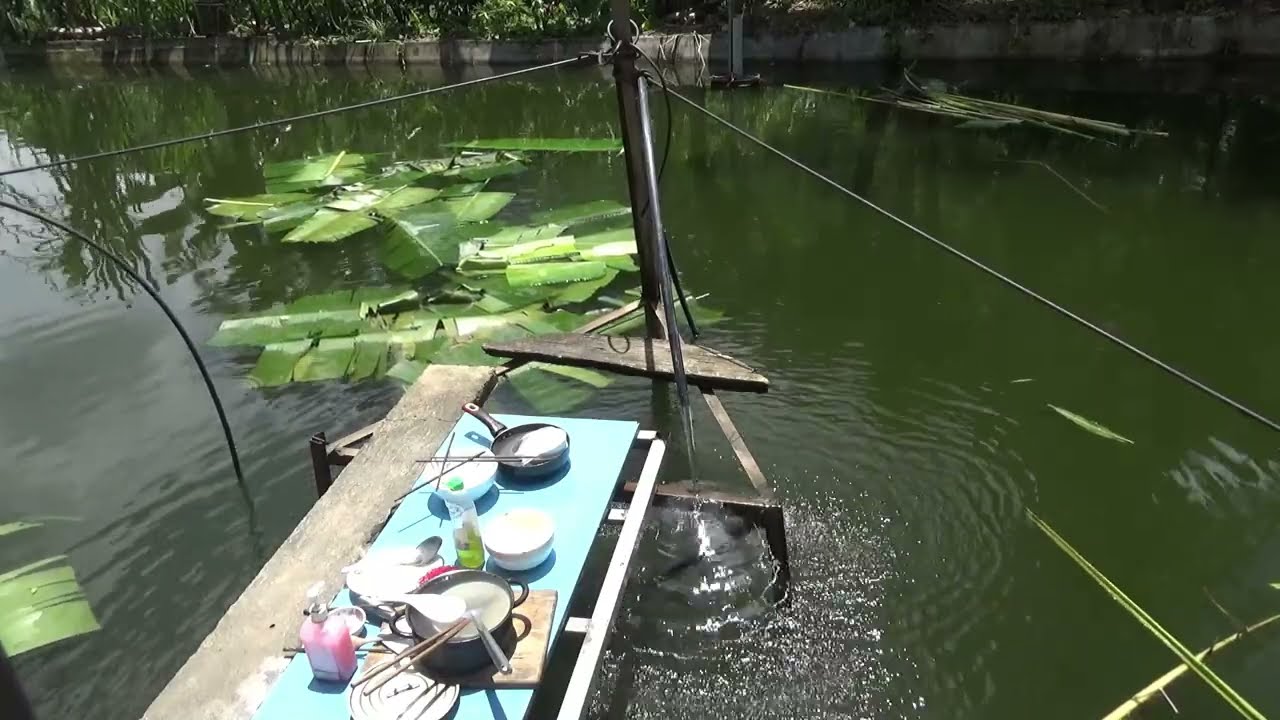The image depicts a man-made canal with deep green water, where broad, tropical-style leaves and branches float on the surface. In the center of the frame, a metal post extends out of the water, with wires running horizontally from it in both directions off the edge of the photo. Attached to the post is a triangular metal base supporting a rectangular platform on which a blue tray rests. This tray holds an assortment of items including pans, pots, bowls, utensils, and cooking supplies, suggesting the possibility of an artist at work or someone preparing a meal. In the background, there is a gray stone or cement wall marked by water lines indicating the previous water level. Greenery with overhanging branches drapes over the top of the wall, adding a touch of nature to the otherwise industrial setting.